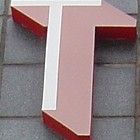In the image, there is a large, 3D block letter "T" affixed to the gray concrete wall of a building. The letter "T" features two distinct shades of red—a darker red on the sides that create a shadowed, three-dimensional effect, and a lighter, pale red on the front surface. Additionally, a smaller, regular-shaped "T" in white is positioned on the left side of the block letter, suggesting part of an incomplete sign or company logo. The detailed textures and dual color tones highlight the visual depth and structural design of the letter against the stark, muted background of the wall.